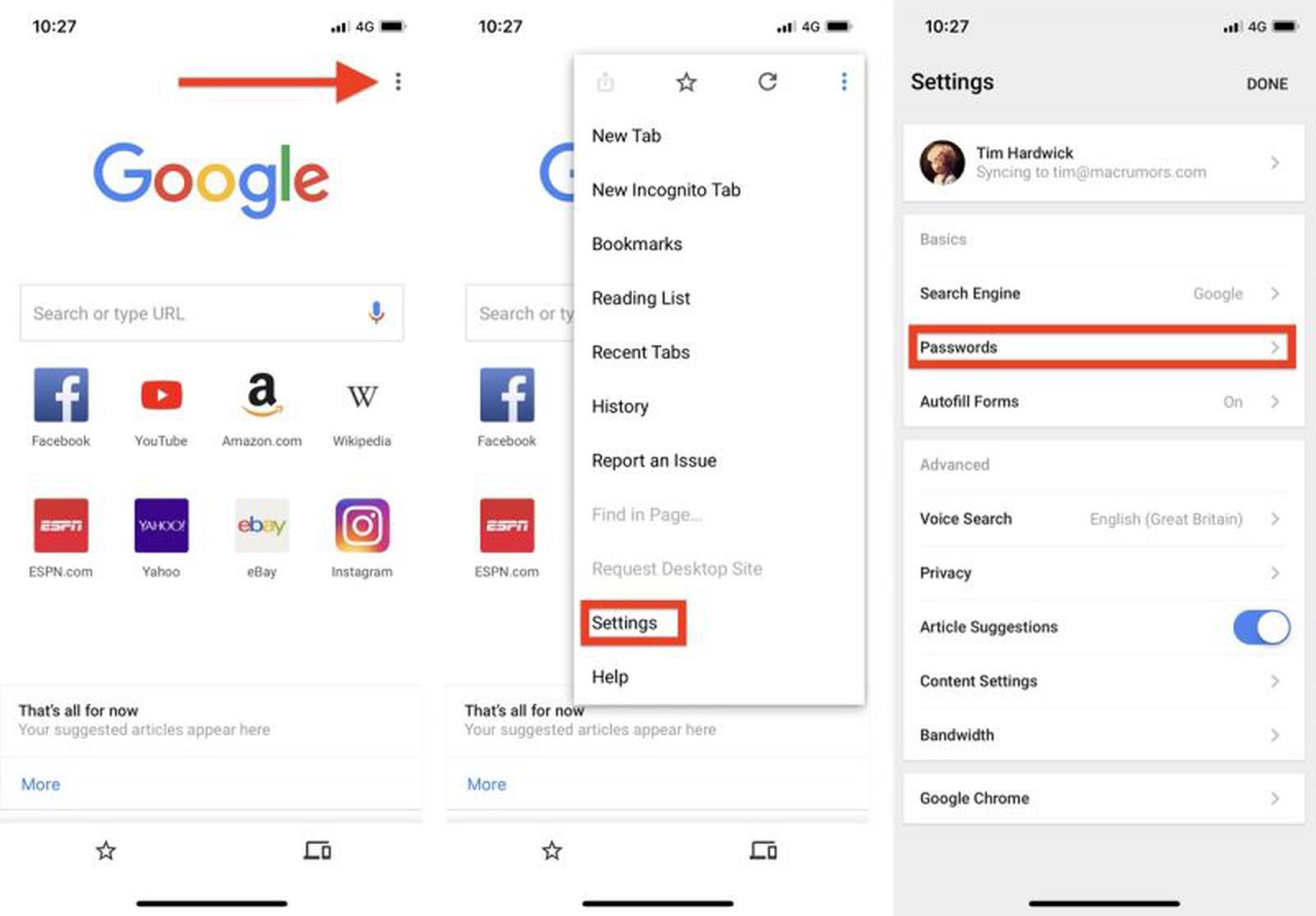Screenshot of a Google Search Page Navigation to Settings

This detailed screenshot captures the sequence of steps on the Google Search app, emphasizing the journey from the homepage to the settings menu. The process begins with the user clicking on the three vertical dots located in the top right-hand corner of the main search page. This action reveals a dropdown menu with several options: "New Tab," "New Incognito Tab," "Bookmarks," "Reading List," "Recent Tabs," "History," and "Report an Issue." Notably, "Find in Page" and "Request Desktop Site" options are grayed out, indicating they are disabled in the current app environment.

Among these options, "Settings" is highlighted with a red box, guiding the user towards the next step. By selecting "Settings," the user is directed to the main settings page, which features their profile at the top. The profile information includes the name "Tim Hardwick" and syncing details to the email "tim@macrumors.com." The settings menu further lists essential preferences such as "Search Engine," "Google Passwords," "Autofill Forms," and "Passwords," with the "Passwords" section also marked with a red box.

This screenshot serves as a step-by-step visual guide aimed at assisting users unfamiliar with navigating from the Google Search homepage to their settings, ensuring they know precisely what to click on at each stage.